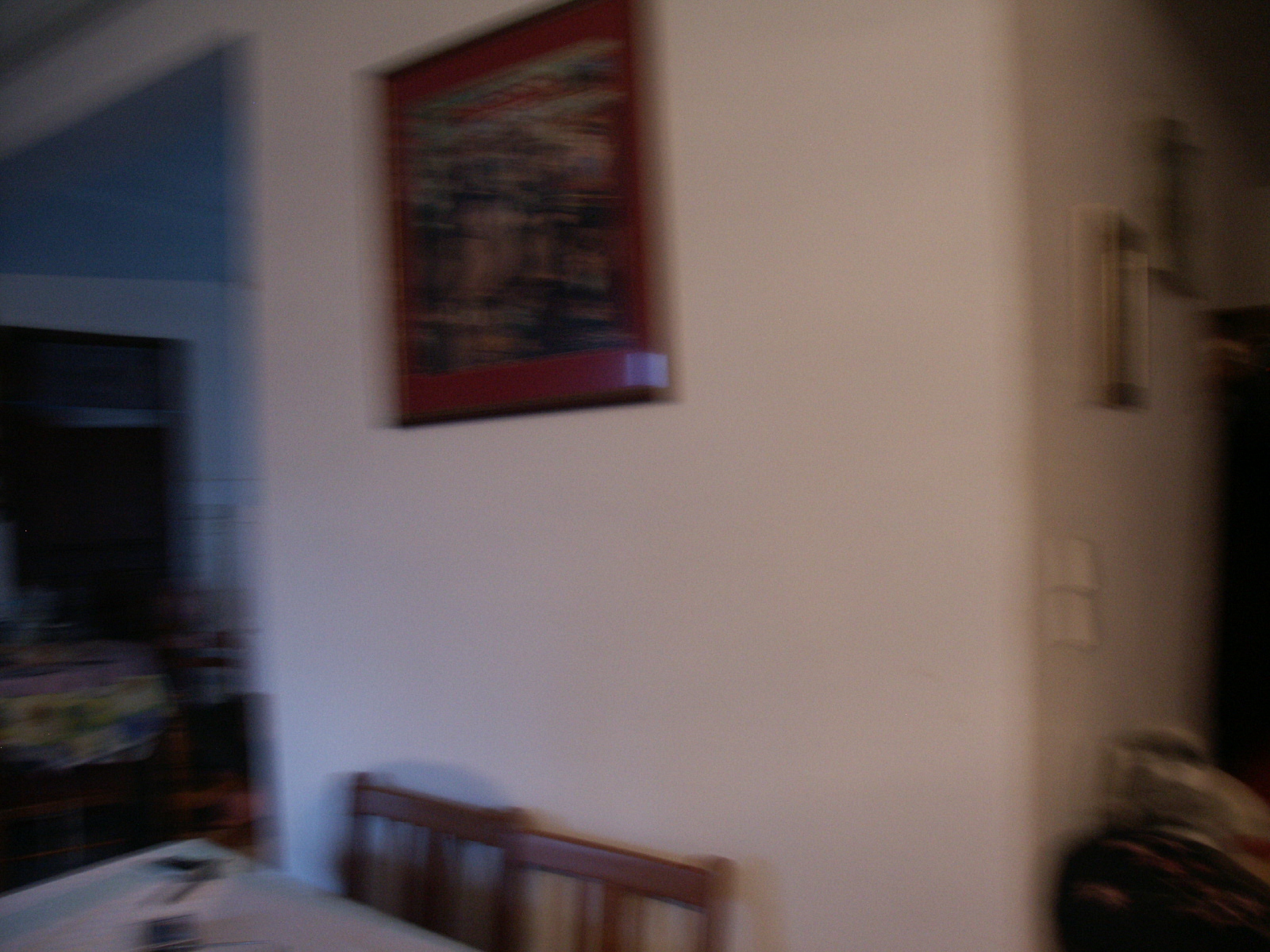In this image, we're looking into a corner of a dining area within a house. The photograph is noticeably blurry, making it challenging to discern specific details. At the bottom, we see the tops of two brown, wooden chairs surrounding a white tabletop. A gray wall takes up a significant portion of the background, adorned with a brown-framed painting that features blurred colors of black, red, and gray. 

To the right, there is a continuation of the white wall, which includes a couple of picture frames and several objects on the ground, along with what appears to be bags or luggage leaning against it. On the left, the wall contains a light switch and a doorway leading to another room. This doorway is large and open, without an actual door to close it off, further adding to the sense of space. The room beyond is even more blurred, making it difficult to identify its contents. There also seems to be a hint of a blue ceiling at the top left corner of the image. The overall impression is one of a spacious but slightly cluttered and lived-in dining area, characterized by neutral and soft-colored walls.